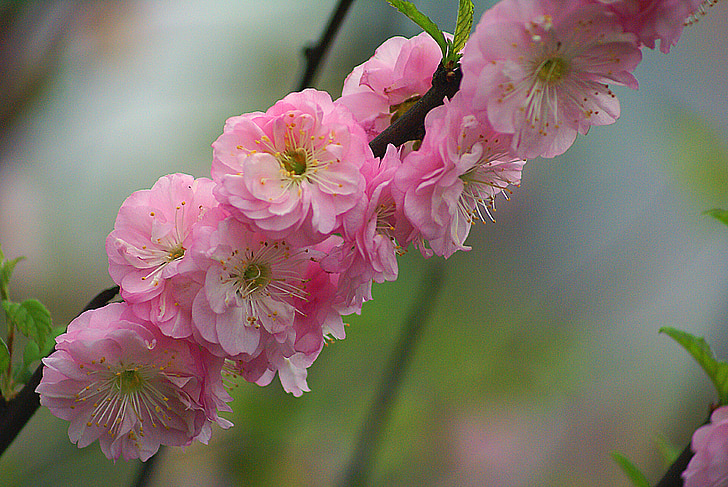This image is a detailed color photograph in landscape orientation, featuring a stem adorned with light pink flowers with white accents, possibly hollyhocks. The numerous blossoms, approximately 10 to 12, are fully bloomed with layers of ruffled petals creating a rounded shape. They extend diagonally from the bottom left to the top right. Each blossom has a greenish-yellow center filled with multiple stamen ending in tiny round beads. Accompanying the pink flowers are a few green leaves scattered along the dark branch, with more visible at the bottom left and top right corners. The background is a blurred mix of green vegetation and dark branches, enhancing the focus on the vibrant flowers while suggesting a lush environment.